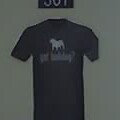This blurred, small photograph (which seems to have a slight green tinge, possibly indicating it's in colour) was taken in very low light. At the center of the image, dominating most of the height, is a black T-shirt with short sleeves. The T-shirt features a white logo at the top, somewhat resembling a sheep or another animal facing left. Below the logo, there are two lines of white text: the upper line appears to be a short word, and the lower line a longer word, though both are too thin and blurry to read. Just above the T-shirt at the upper edge of the photo, there is a greyish-black, squarish object with what looks like two round elements flanked by a couple of square elements on either side, adding an enigmatic touch to the scene.